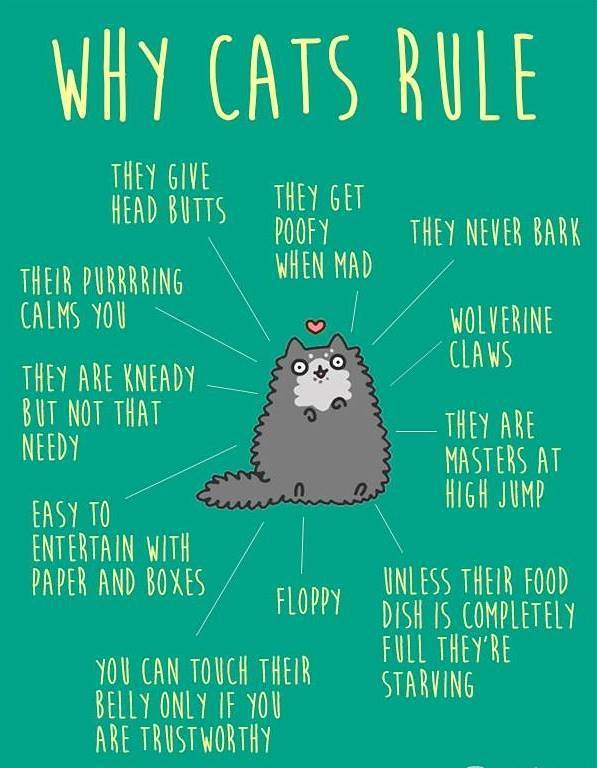The image features a detailed infographic titled "Why Cats Rule," placed at the top in lemon-colored ink against a green background. At the center of the infographic is a cartoon drawing of a grey cat with short legs, sitting upright. Above the cat's head is a red heart. Surrounding the cat are various text highlights in yellow, listing charming and unique behaviors of cats: they give headbutts, get poofy when mad, never bark, have wolverine claws, are masters at high jumps, believe they are starving unless their food dish is completely full, are floppy, allow belly touches only if you are trustworthy, are easily entertained with paper and boxes, are needy but not excessively so, and their pawing calms you. The text playfully characterizes the endearing quirks that make cats beloved pets.